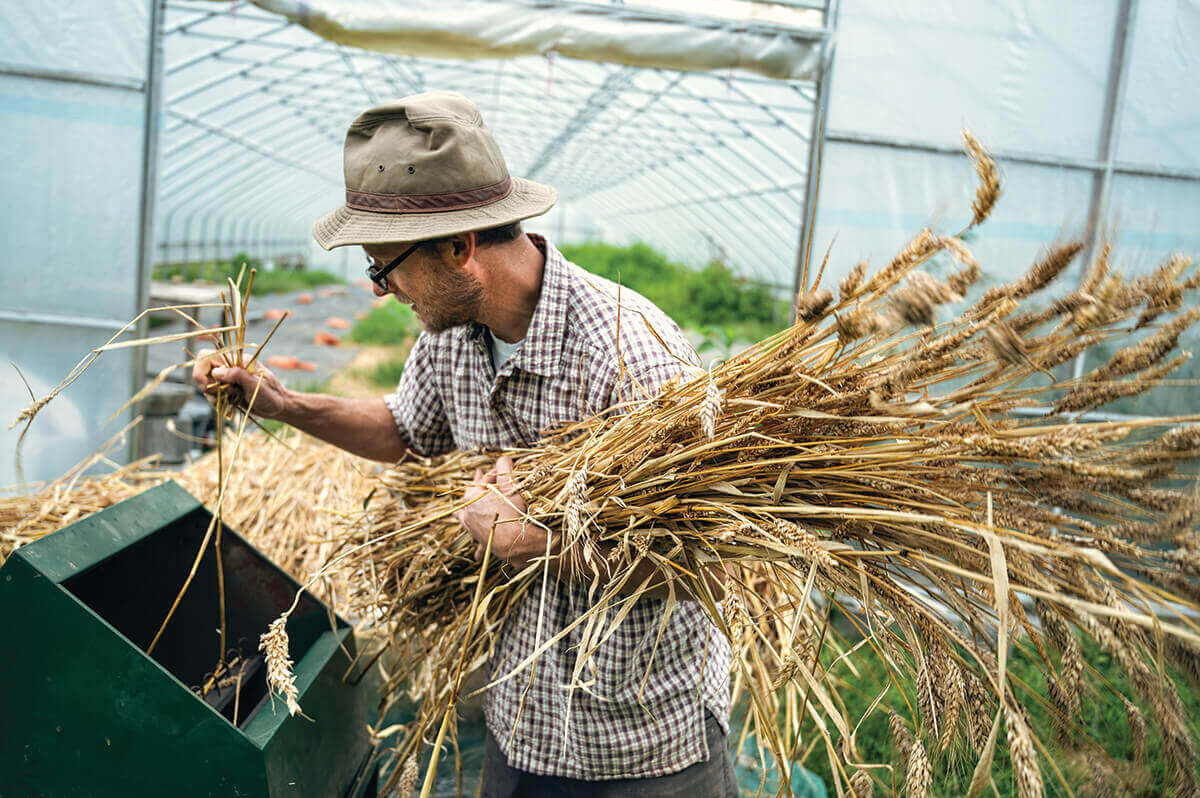A bearded man, possibly a farmer, is standing in front of a large greenhouse with rolled-up plastic doors, feeding an armful of brown wheat stalks into a green metallic machine, which appears to be a shredder or chipper with visible teeth. He is wearing a short-sleeved, plaid brown and white shirt over a white T-shirt, along with gray pants and a khaki-colored sun hat. He completes his look with dark-framed glasses. The greenhouse behind him features a walkway with green plants and pink objects visible inside, with additional greenery present in the background to the right. This scene captures the man engaged in the meticulous task of processing the wheat stalks, though the exact nature of the operation remains unclear.